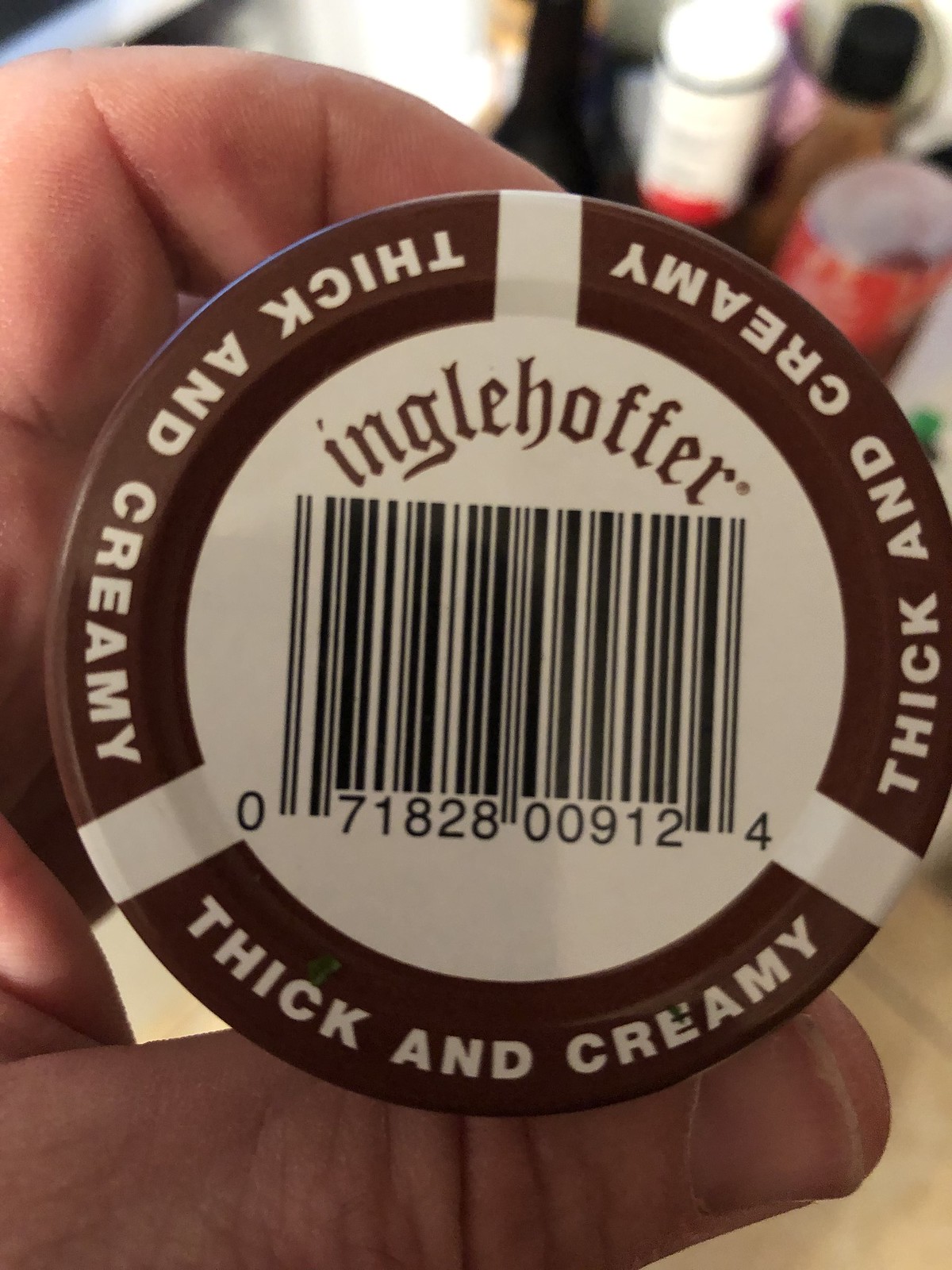In the image, a hand is shown holding a brown label that prominently features the words "thick and creamy" and the brand name "Engelhofer." The person holding the label appears to be of Caucasian descent, with their thumb and index finger visibly gripping the object. The label, which might be from a bottle rather than a beer, includes a barcode on its back. The background of the image is slightly out of focus, revealing what appear to be either drinks or cans. A white surface, possibly a table where the person may be resting their elbow, is also visible in the scene.